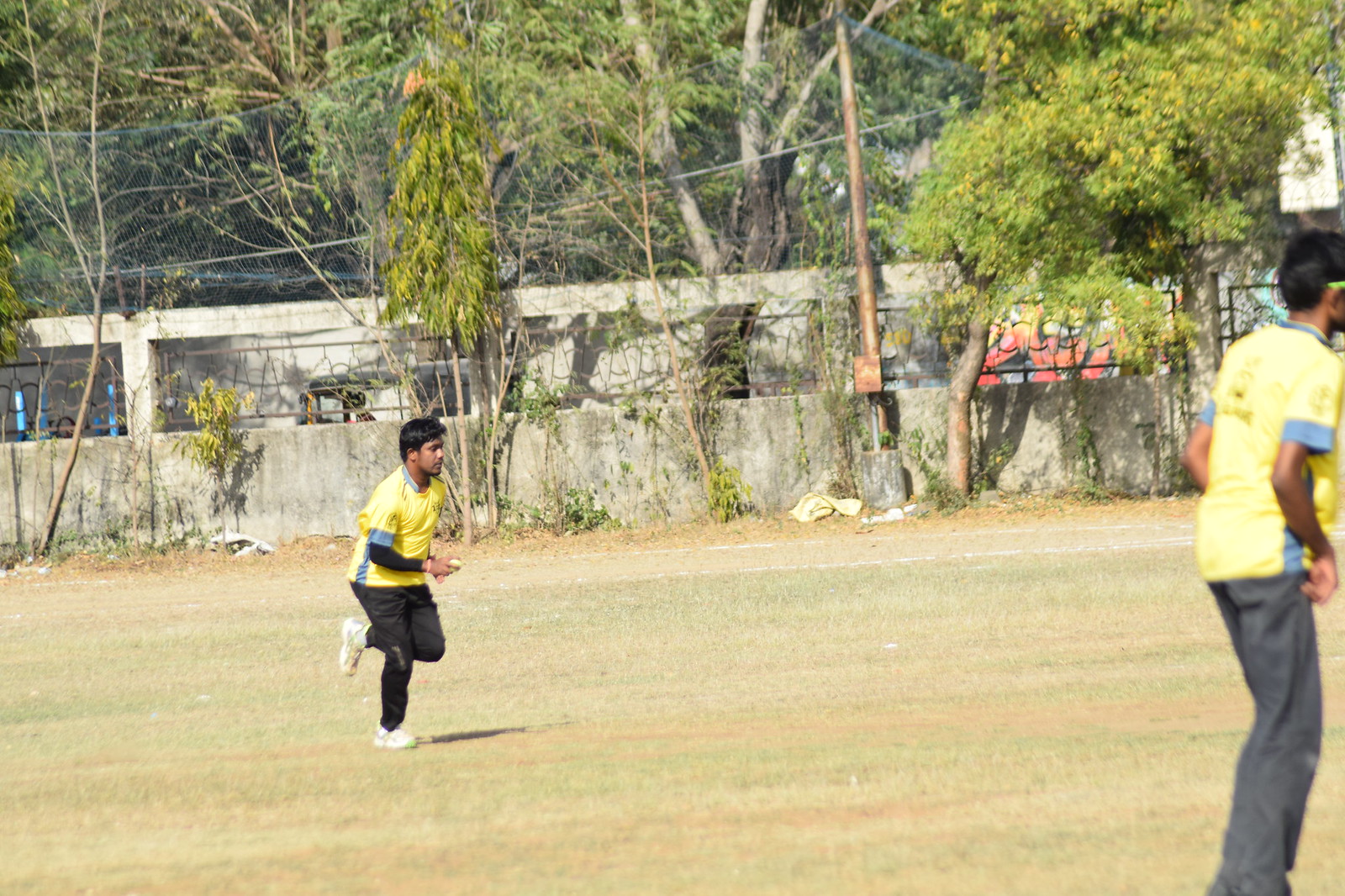The image captures two men running across a dehydrated field with scattered green patches. Both men have dark skin and short black hair, suggesting they may be of Indian descent. The foreground shows a man in motion, wearing black long pants, white shoes, and a yellow shirt layered over blue and black undershirts, featuring a blue stripe under the armpit. Another man stands on the far right, clad in a similar yellow shirt with green accents and light gray pants, facing away from the camera. The field is surrounded by a high stone wall topped with a metal grate, beyond which several buildings are visible. Trees, some green and some brown, and power lines line the perimeter of the field, adding to the sense of a dry, arid environment. The scene suggests they may be engaged in a sport, possibly baseball or soccer, indicated by their matching sporty attire and the fabric-covered fence around the field.